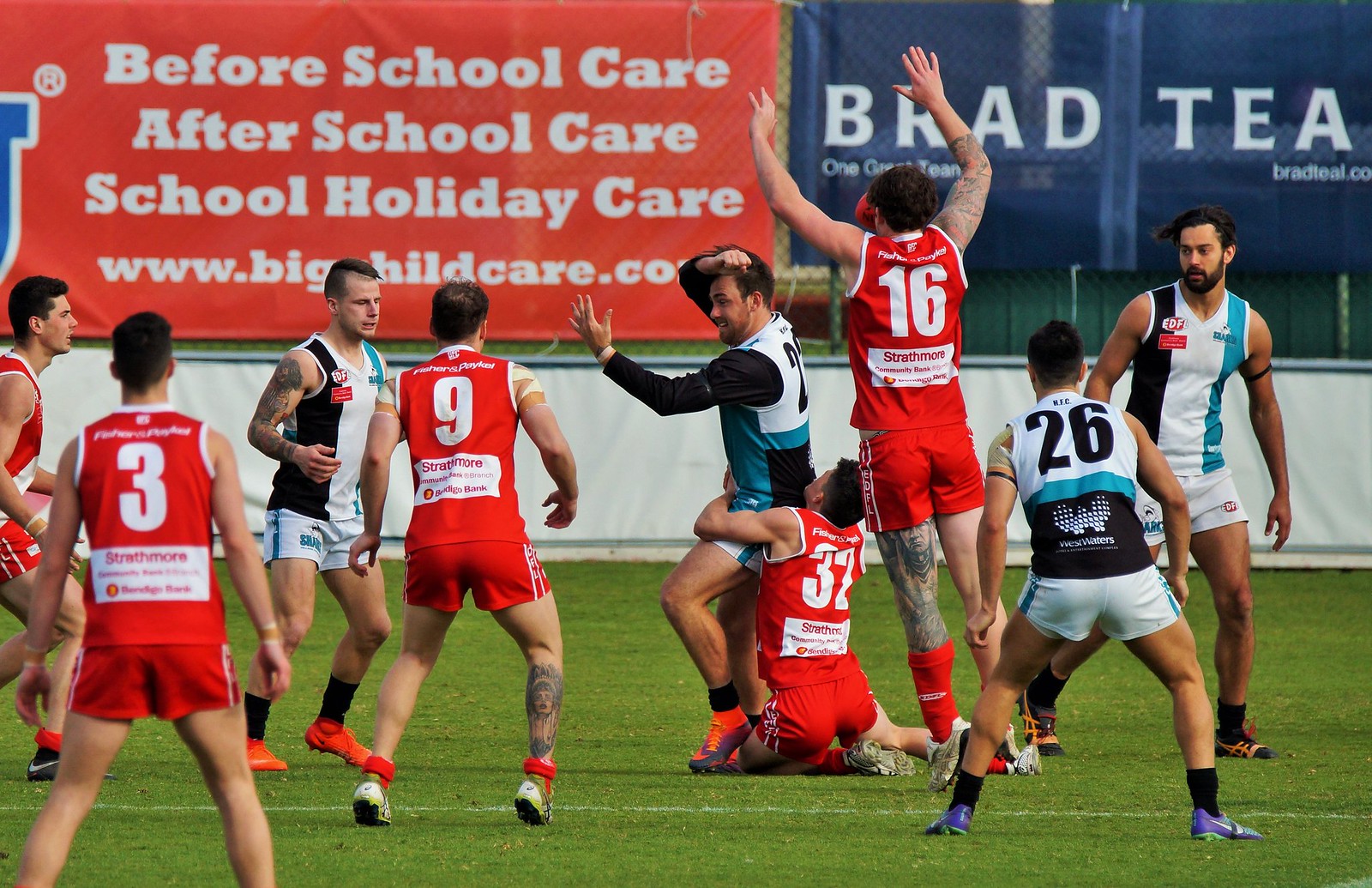In the vibrant image capturing a dynamic sporting event on a soccer field, it appears that a rugby match is in full swing. The athletes, dressed in distinct team uniforms—one in red with white numbers and accents, the other in white, blue, and black—are intensely engaged in the game. Central to the photograph, a player in red, number 32, is seen fervently tackling his opponent in black and white, who has just tossed the ball upwards, perhaps in a last-ditch effort to pass before hitting the ground. Surrounding this pivotal moment, other players react: a red-suited player with number 3 and another with number 9, both focused and poised for the next move, while others in white, black, and blue jerseys position themselves strategically. Above the action, various sponsors' banners—promoting services like "Before School Care, After School Care, School Holiday Care," and brands such as "Brad T"—line the field's perimeter, adding a backdrop of commercial color and support. A white fence and assorted billboards stretch across the background, framing this intense moment of the rugby match.